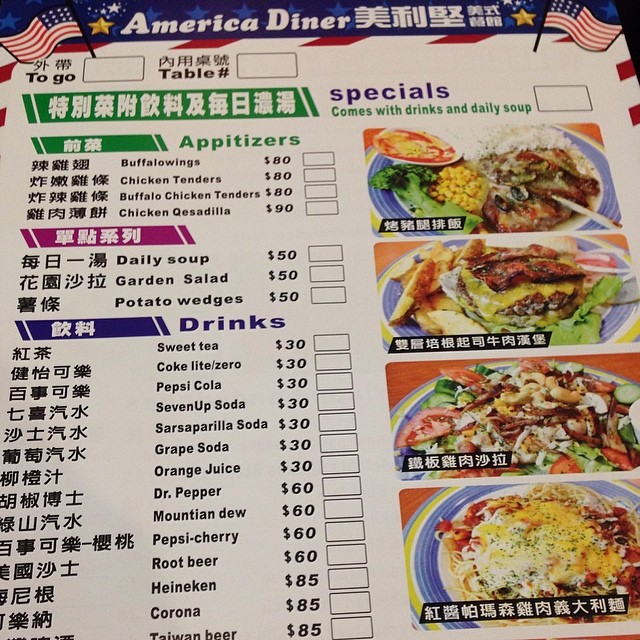This is a vibrant and detailed photo of an American diner menu found in Asia, reflecting a lively fusion of American and Asian influences. The backdrop of the menu is strikingly blue, adorned with white stars and a couple of gold stars, evoking a patriotic American theme. Complementing this are two American flags, one positioned on the left and the other on the right side of the menu.

At the top of the menu, there are designated boxes, one labeled "To Go" and another for the "Table Number," each accompanied by Asian characters. A section below announces the specials, which include drinks and daily soup. The menu features an array of food pictures, each labeled exclusively with Asian characters. Among these images, a hamburger and what appears to be enchiladas can be identified, along with dishes that include broccoli, corn, and rice.

On the left side of the menu, several sections are organized, starting with a green-labeled "Appetizers," which lists various starter options. The middle section is presented only in Asian characters, while the bottom section titled "Drinks" offers an extensive list of beverages. This drinks list, written in a royal blue font, encompasses both alcoholic and non-alcoholic options, catering to varied preferences.